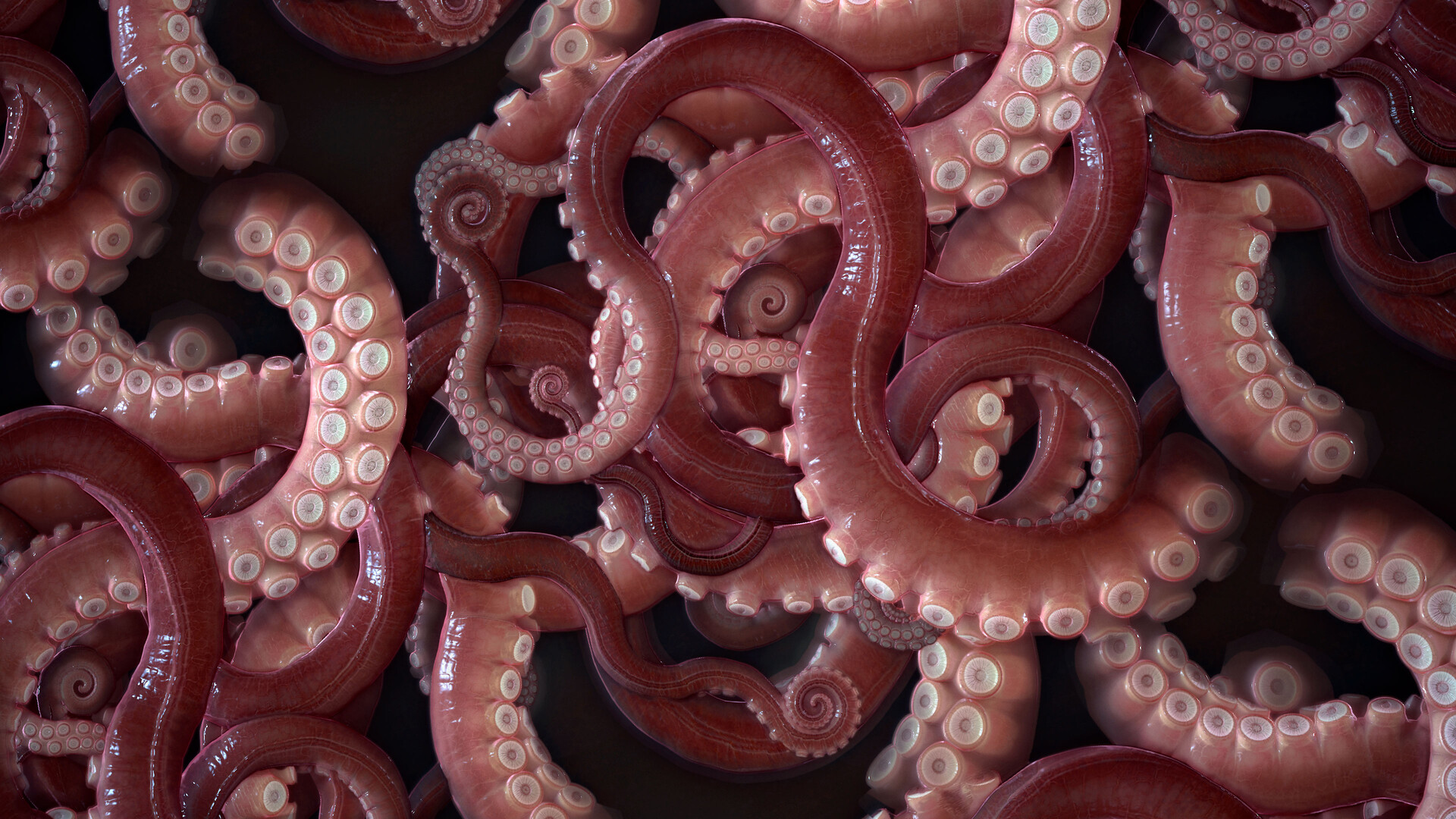This detailed close-up image, possibly sourced from an educational textbook or informational magazine about marine life, captures a dense intertwining of numerous octopus tentacles, potentially belonging to several octopi. The tentacles, numbering over twenty, are an intricate mass, twisting in and out over one another against a stark black backdrop. The tops and sides of these squiggly appendages are colored in a rich maroon or dark red, while the undersides feature a gradient from white to light pink. White suction cups, arranged in pairs all along the bottom of the tentacles, add to the elaborate texture of the scene, highlighting the extraordinary details of these fascinating sea creatures.